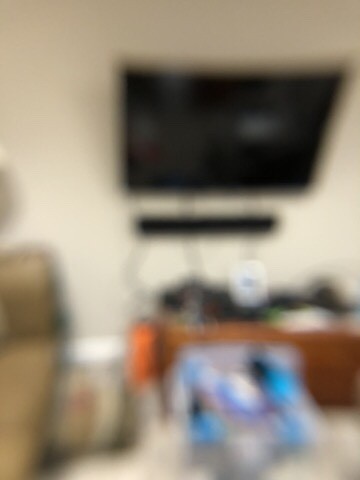A highly blurry image taken inside a house, possibly the living room or den. The focal point is a wall-mounted TV, which remains turned off with a similarly blurry and unidentifiable image on the screen. Below the TV, a soundbar is visible, with cables trailing down from both the TV and soundbar. Beneath these, a cluttered stand or dresser holds various objects, including a white device that could be a modem, router, or dehumidifier, alongside a piece of cloth. To the right side of the image, there's what appears to be a chaise lounge. In the foreground, there is an indistinct, multicolored object in shades of blue, gray, and white. The overall image suffers from significant blur, making finer details difficult to discern.